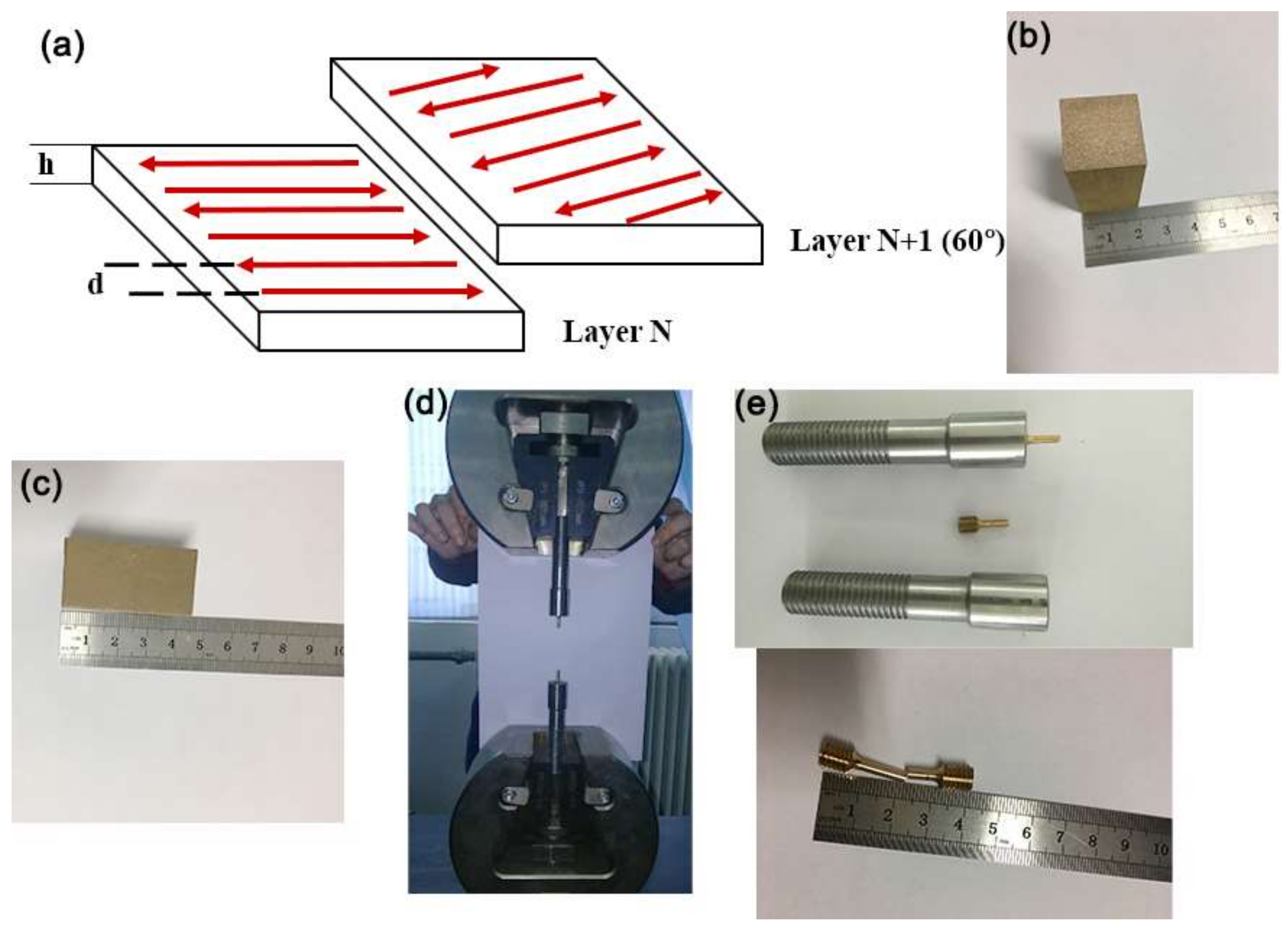The image is a detailed collage of diagrams and photographs centered around measurements and labeled machinery parts, set against a white background. It features five distinct sections labeled A through E, each showcasing different elements.

- **Section A** illustrates two white blocks with red arrows, positioned to slide together, and includes annotations "Layer N" and "Layer N + 1 (60 degrees)."
- **Section B** depicts a metal ruler next to a rectangular block.
- **Section C** shows a block laid on its side next to a ruler measuring close to 5 inches.
- **Section D** includes what appears to be a piece of machinery within a room, possibly featuring a heater on the wall, and has someone’s hands positioned on either side.
- **Section E** displays several silver bolts and a metal ruler measuring brass couplings or screw-like objects.

Collectively, the image appears to be instructional, likely detailing steps or measurements related to assembling or inspecting machinery parts.